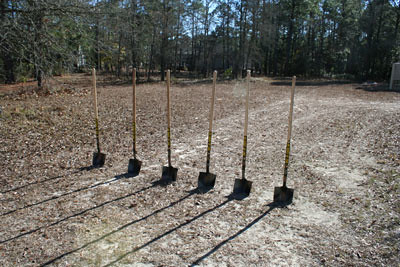This exterior photograph, taken on a bright, sunny day, showcases a dirt field surrounded by a green tree line and a blue sky peeking through the foliage. Central to the image are six shovels arranged side by side, standing upright with their blades embedded in the tilled soil. The handles of the shovels, likely made of wood, cast long, distinct shadows in front of them, creating a striped pattern on the ground. In the background, beyond the cleared and muddied area, a wooden fence separates the field from the forested area. The sunlight, originating from the upper right of the frame, enhances the natural lighting and the clarity of the shadows.